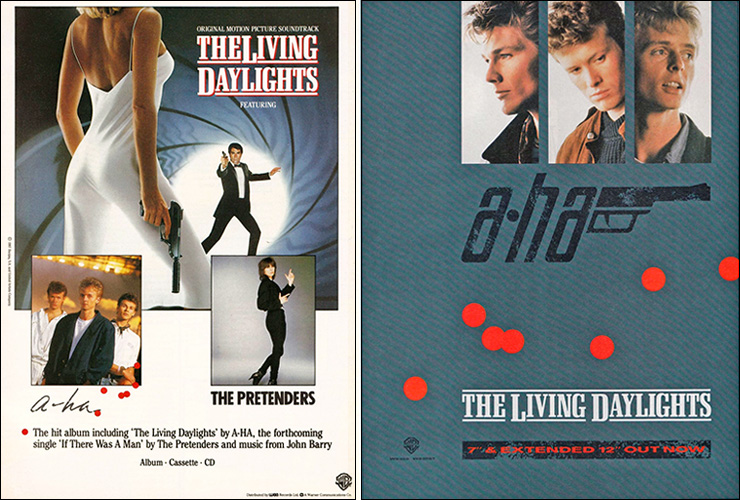This composition features a dual-poster advertisement for the James Bond movie "The Living Daylights" and its soundtrack, prominently highlighting the involvement of the band A-ha. 

On the left side is the movie poster. At the top right, in white lettering, it reads "The Living Daylights." The focal point is a striking image of James Bond emerging through the iconic gun barrel, aiming his weapon at a blonde woman seen from behind. She is clad in a see-through, white spaghetti strap dress, also holding a gun. Below this visual, a black rectangle lists "The Pretenders" and includes an image of their singer. Next to it is another picture showcasing the band A-ha, with details about songs from the movie's soundtrack. Prominently mentioned is the hit album, featuring "The Living Daylights" by A-ha, the forthcoming single "If There Was a Man" by The Pretenders, and music composed by John Barry. The poster notes availability in album, cassette, and CD formats.

The right side of the composition focuses on the band A-ha. It features a blue background adorned with scattered red polka dots. The top section displays three individual photos of the band members. Below these images is the band’s logo, stylized to resemble the 007 logo with a gun barrel motif, and the text "A-ha" in black. At the bottom, it announces in white letters, "The Living Daylights," along with "extended 12-inch out now" in red.

Altogether, this detailed and visually engaging advertisement underscores the collaboration between the James Bond franchise and A-ha, promoting the soundtrack and the film vividly.